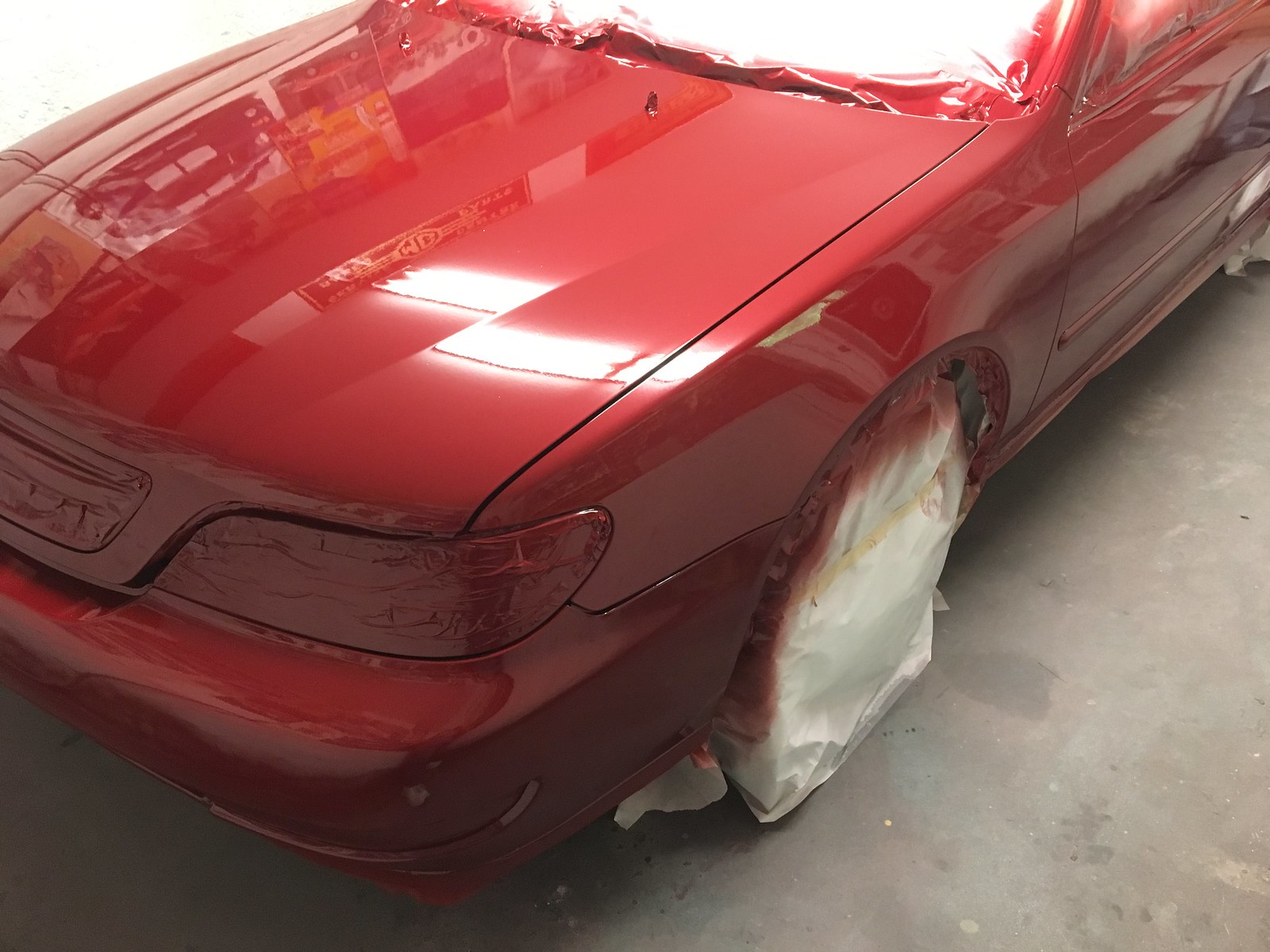This image is a detailed indoor photograph showcasing a bright red car in the process of being painted. The vehicle, parked on a gray concrete floor, is seen from a three-quarter view, revealing the front hood, left fender, and partial left door. The car, likely an older model from the early 90s, gleams under the overhead fluorescent lights, with reflections clearly visible on its glossy surface. The windshield, headlights, grille, and driver-side tire are meticulously covered with white plastic and masking tape to protect them from overspray. The windows are also taped up and masked with white plastic. No text or print is present in the image, and the lighting creates a slightly darker ambiance in the left foreground, contrasting with the brighter right side. The scene suggests the car is in a paint booth, evidenced by the uniformity of the masking and the precise application of bright red paint.